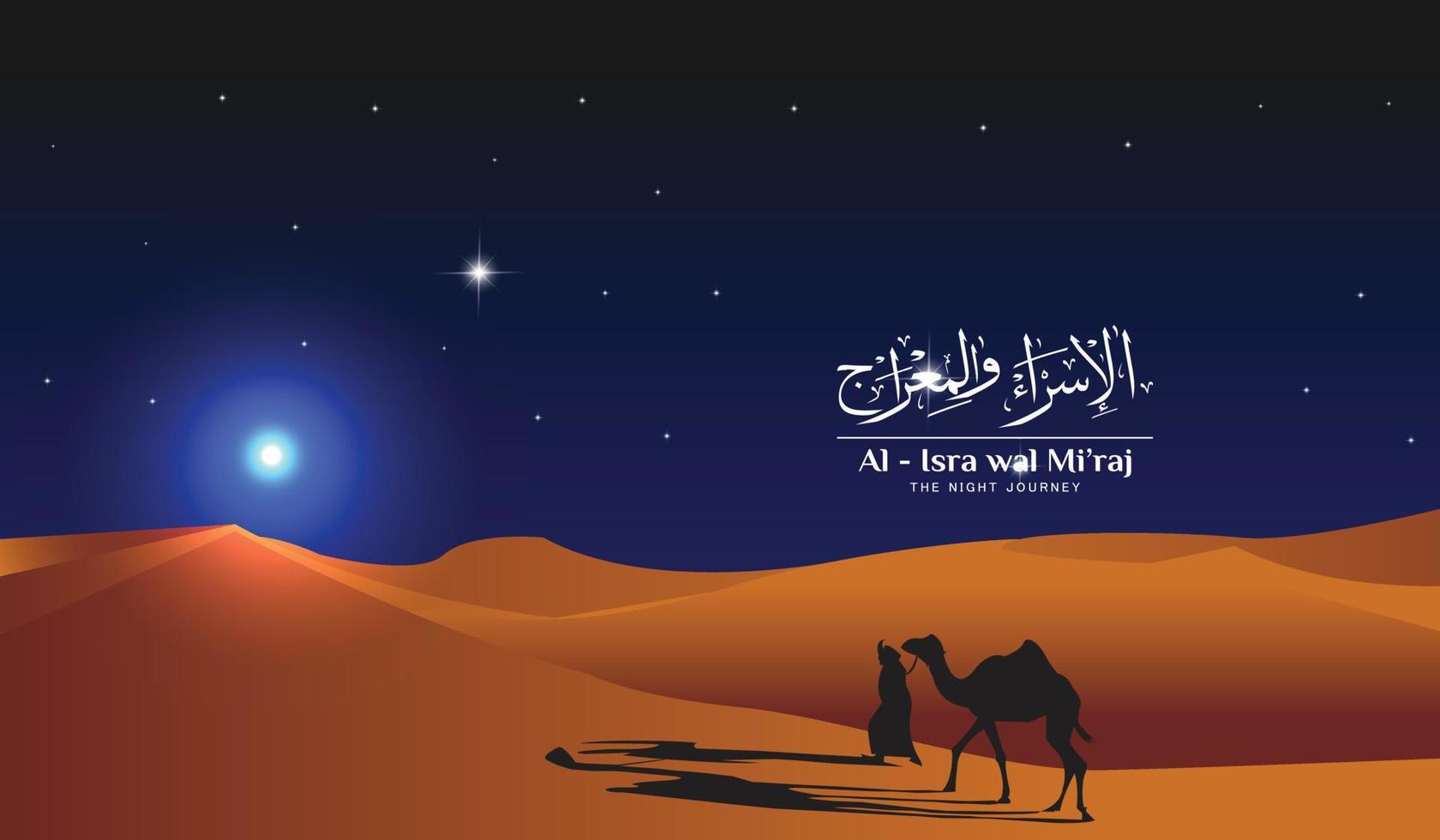This is an animated poster in a horizontal landscape orientation titled "Al Isra Wal Miraj," which translates to "The Night Journey." The scene depicts a man walking a camel through an orange-hued desert with varied terrain and sand dunes. The desert is painted in red and brownish shades, occupying the lower third of the image. Above, the night sky dominates with a dark purple hue. A full moon shines brightly on the left side of the sky, near the horizon, and nearby stars fill the backdrop, including one particularly bright star positioned to the right and above the moon. Arabic writing adorns the right third of the poster, adding a cultural authenticity to the visual narrative.